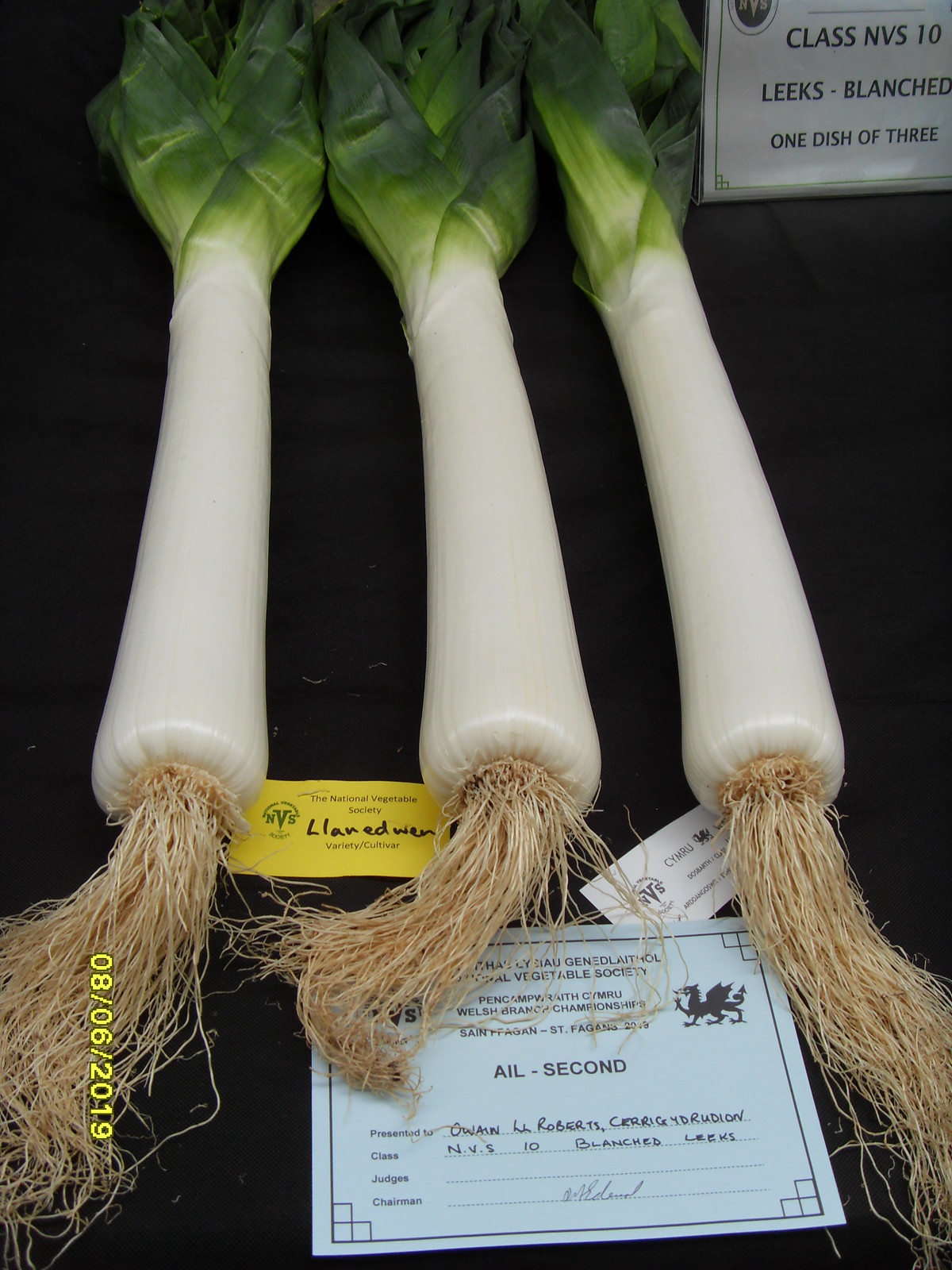In this image, a variety of objects are meticulously arranged on a black table, with the focal point being a trio of large, freshly-blanched leeks positioned diagonally from the bottom left towards the center of the image. The leeks, with their white stalks and vibrant green leaves, exhibit long roots extending from their base. In the top right corner, there is a sign labeled "Class NVS 10 Leeks Blanched One Dish of Three," indicating the category of the competition. A second place card is prominently displayed at the bottom of the image, signifying the leeks' awarded position in the contest. The date "08-06-2019" is visible in the bottom left corner, suggesting the event took place on June 8th, 2019. The colors in the image include shades of black, white, green, gray, light blue, and tan, creating a visually striking composition. The setting appears to be a competitive exhibition, likely indoors or possibly in an enclosed outdoor area dedicated to showcasing vegetables.